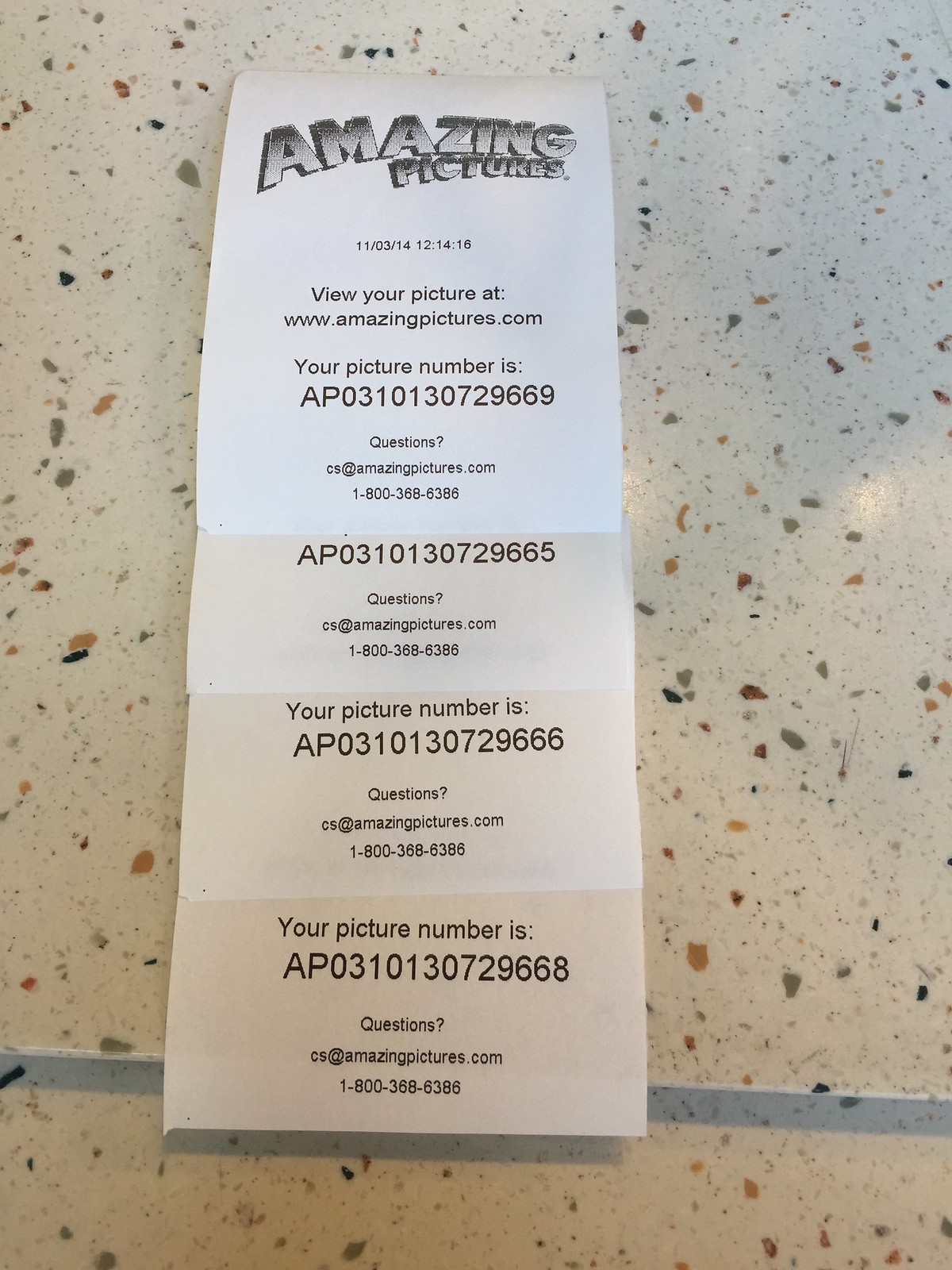This is a detailed photograph of a long, white receipt placed on a speckled white surface. The surface features distinct speckles in various shades including black, light brown, orange, gray, and red, giving it a marble-like appearance. At the top of the receipt, there's a grayscale logo in black and gray bubble font that reads "amazing pictures." Directly below this logo, the date of purchase, "11-03-14," and the time "12:14:18" are printed. Additionally, the receipt instructs the viewer to access their picture online at "www.amazingpictures.com." The unique picture number, "AP0310130729669," is provided and this number is repeated multiple times throughout the receipt. Towards the bottom, the receipt offers contact information for questions, including an email link and a phone number, "1-800-368-6386." The receipt text is primarily in black, contributing to a clear contrast against the white paper and speckled background.